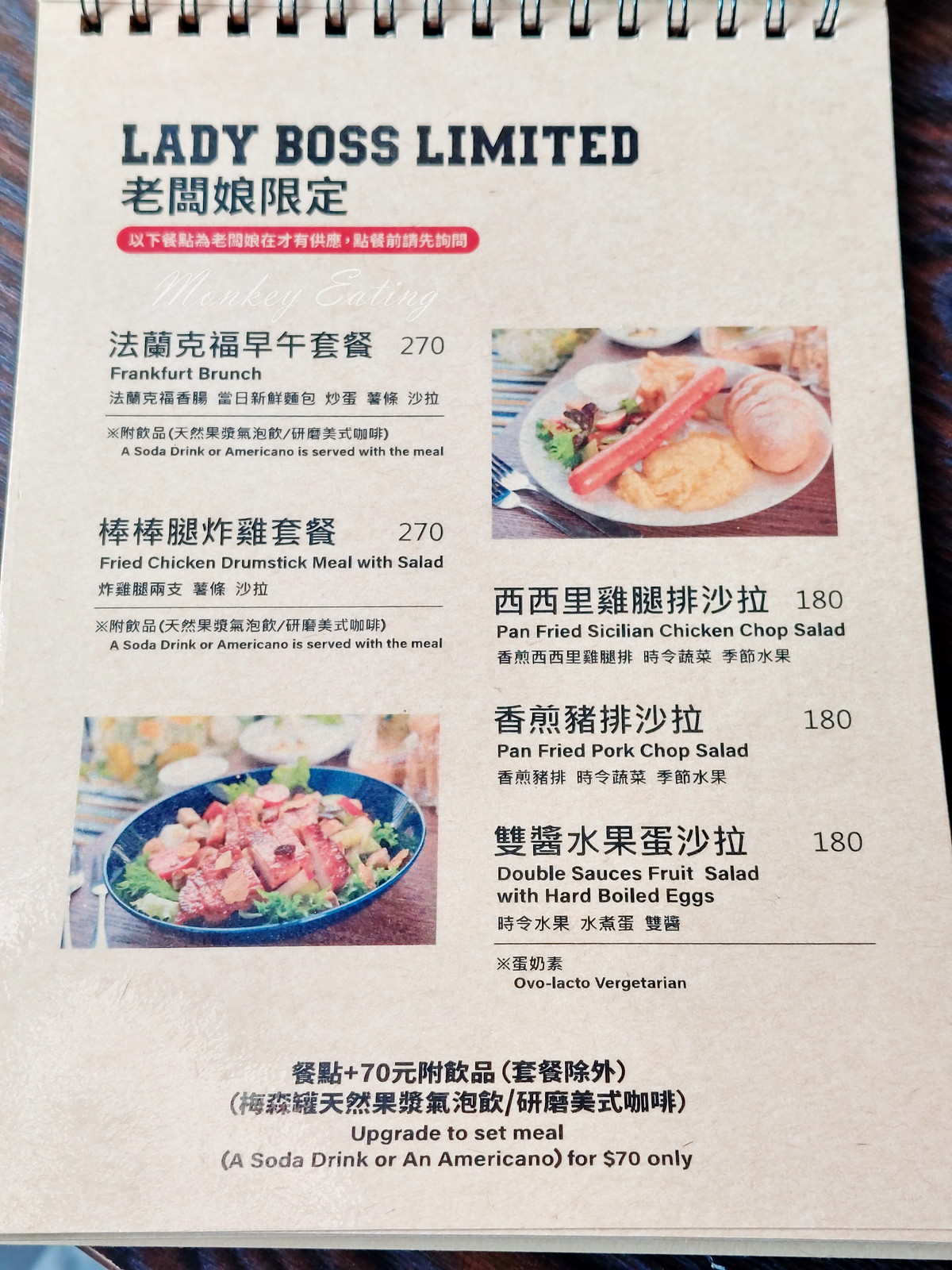This image captures a detailed section of a menu from a restaurant named "Lady Boss Limited," as indicated at the top of the page. A segment of Chinese text is also present, though its meaning is not discernible without knowledge of the language. Centered on the menu, the phrase "monkey eating" is prominently displayed in a white font, although its relevance remains unclear. 

The menu items featured include a variety of combinations priced affordably. The "Frankfurt Brunch" is listed at $270 and comes with a choice of either a soda drink or an Americano. Another offering is the "Fried Chicken Drumstick Meal with Salad," also priced at $270, which includes the same beverage options. For $180, customers can enjoy a "Pan-Fried Sicilian Chicken Chopped Salad" or a "Pan-Fried Pork Chopped Salad." Additionally, a "Double Sausage Fruit Salad with Hard-Boiled Eggs" is available for $180.

Accompanying the menu is an illustrative pair of food photographs. The first image shows a vibrant chicken salad served in a blue bowl. The second photo depicts a detailed arrangement of food on a white plate, including sausage, rice, hard-boiled eggs, and a salad, with two forks placed beside the dish. These visuals provide a tempting preview of the meals offered.